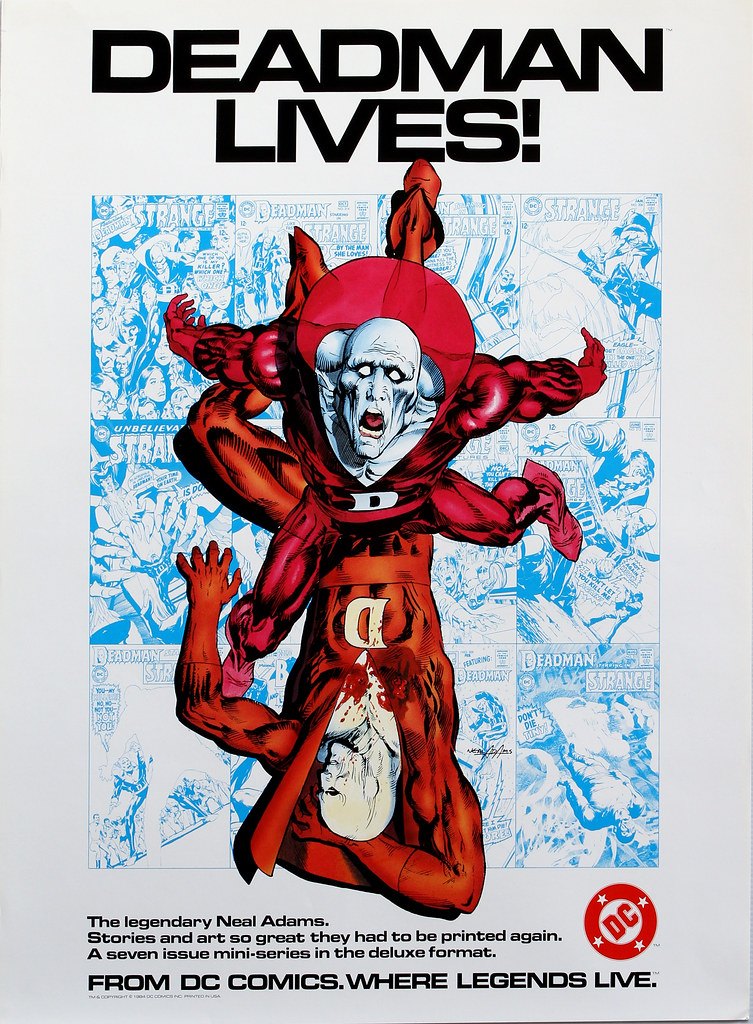This vertical rectangular image appears to be a comic book cover or poster, showcasing a striking and grotesque illustration against a blue and white background. At the top of the image, bold black letters proclaim, "Dead Man Lives!" Below this text is a vividly detailed depiction of a monstrous figure adorned in a red bodysuit with a white capital D on its chest. The creature, with a grotesque white face resembling a goblin and an open mouth revealing a red tongue, is portrayed both right side up and upside down, giving it an almost octopus-like appearance with multiple limbs extending outwards. The background features intricate, blue illustrations that add depth and a sense of chaos. A white border frames the entire composition. 

In the lower left-hand corner, black text reads, “The legendary Neil Adams. Stories and art so great that they had to be printed again. A seven-issue miniseries in the deluxe format from DC Comics, where legends live.” In the lower right-hand corner, a red circle contains the DC Comics logo, adding a mark of authenticity and prestige to the piece.